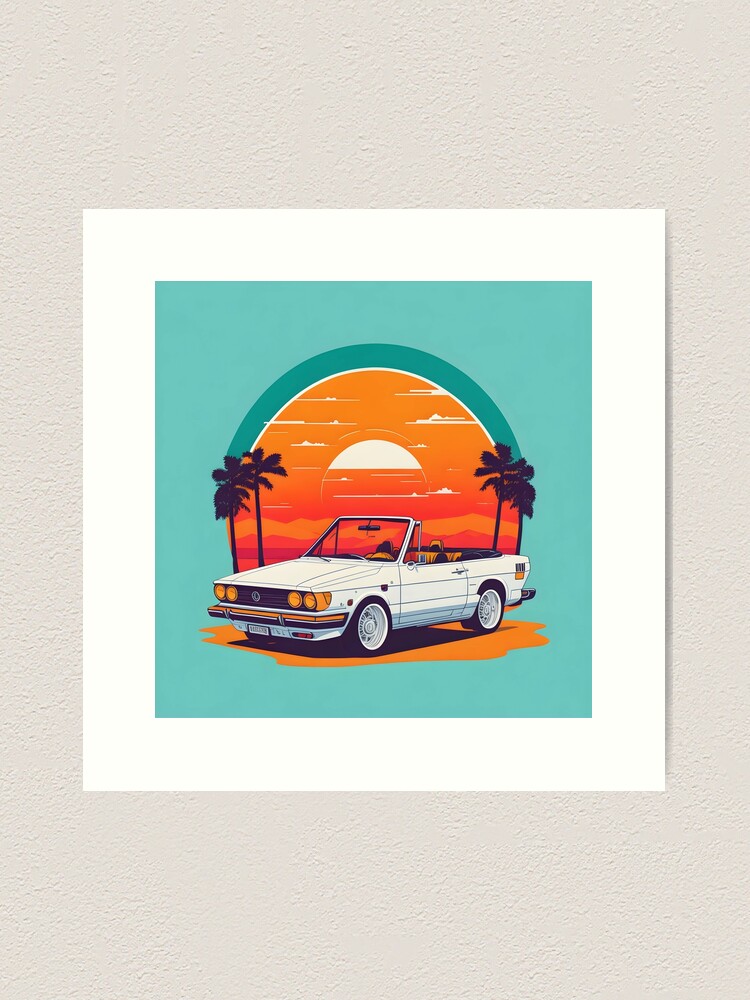The image features a vividly detailed painting set on an off-white textured background. The artwork is framed within a white outer border and a blue inner border. The central focus of the piece is a vintage 1980s-style white convertible coupe with a boxy body and its top down, facing left. This convertible, showcased with an orange bumper, orange interior, and four orange headlights, is posing against a scenic sunset. The backdrop encompasses a radiant orange sky transitioning to red hues, with the white sun partially hidden by horizontal white clouds.

Flanking the convertible are four tall, black silhouette palm trees—two on each side, adding a tropical touch to the scene. The entire sunset and car are enveloped in a small, circular teal background, enhancing the vibrancy of the scene. This vivid depiction is a striking homage to a nostalgic era, encapsulating the essence of a sunlit horizon with palm trees and a classic car in one harmonious, captivating frame.